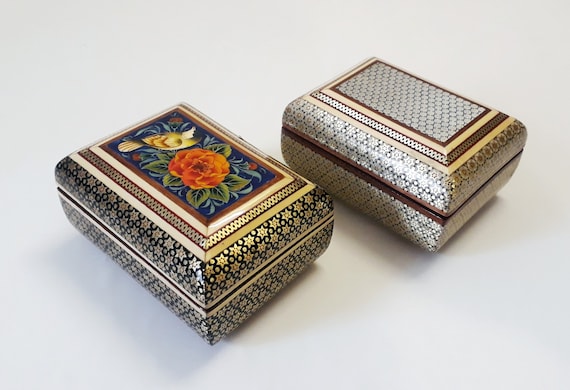In this image, there are two ornate boxes placed at an angle next to each other on a light gray, almost white, background. Both boxes are nearly cuboidal but feature slightly curved corners, resembling a pillow-like design with a clearly visible seam in the middle, indicating where the lid meets the base.

The box on the left boasts a vibrant and intricate design. Its top center showcases a detailed painting of flowers and leaves, with the flower depicted in orange and the surrounding leaves in green, all set against a blue background. Surrounding this central painting are multiple borders: a brown border, followed by a green one, then another brown border with fine designs, and finally another green border. The body of the box is adorned with golden star shapes dispersed across an elegant black background.

In contrast, the box on the right features a more subdued design palette. Its body has a cream-colored field with star-shaped patterns, and the top is decorated with silver circles. The primary colors on this box are shades of cream and brown.

The setting creates a minimalistic yet sophisticated backdrop, emphasizing the ornateness and design intricacy of the boxes.